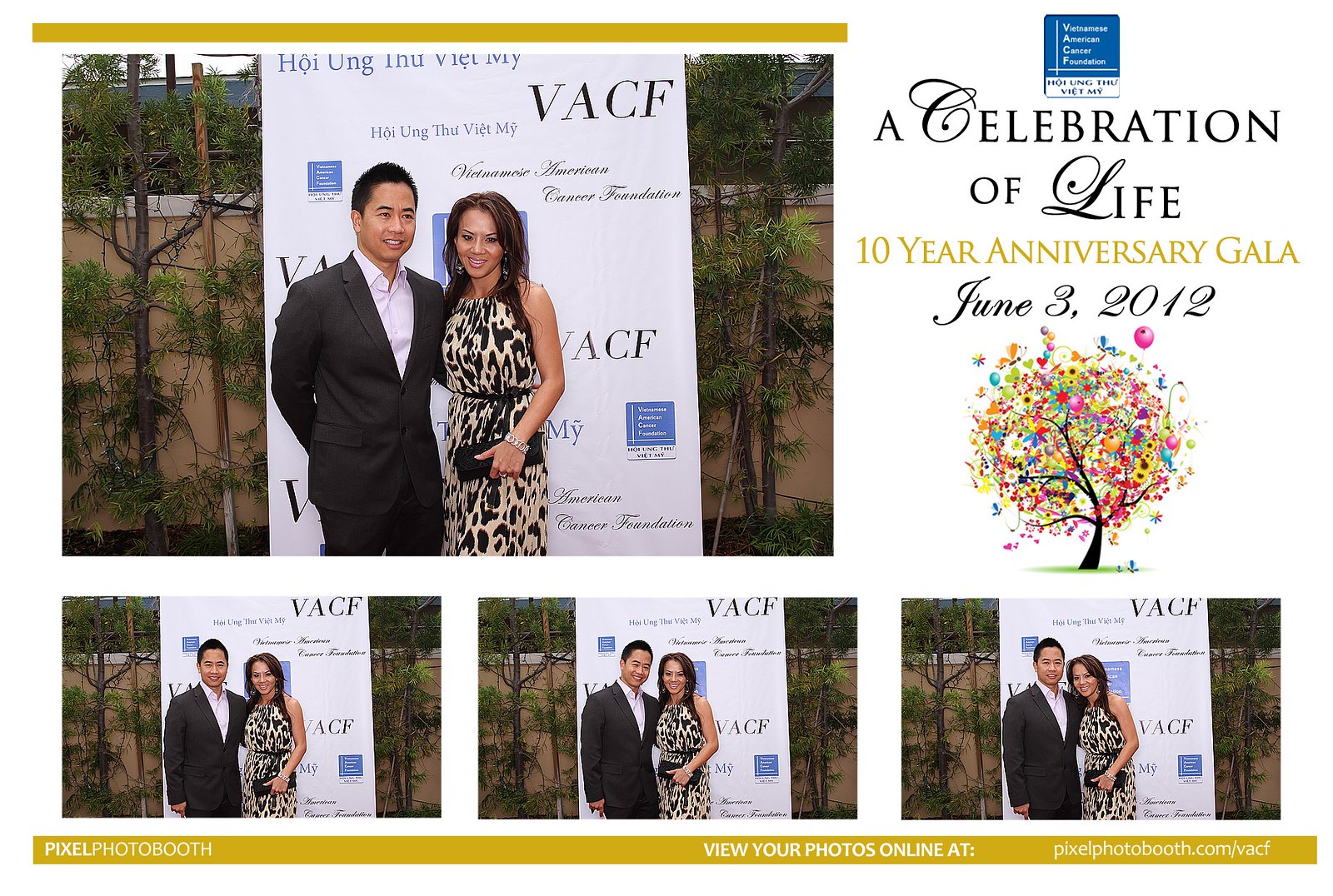The graphic consists of a series of four photos from the "Celebration of Life 10-Year Anniversary Gala" held on June 3, 2012, organized by the Vietnamese American Cancer Foundation (VACF). The couple in the photos, who appear to be of Asian descent, are dressed formally. The man is wearing a dark-colored suit with a white shirt, but no tie. The woman is adorned in a black and gold animal-print dress, complemented by a black clutch bag and a beautiful bracelet. They are posing against a backdrop featuring a white screen listing the event sponsors and a decorative drawing of a tree with colorful leaves and flowers. Behind them, small trees and a brick wall are visible. Additionally, the corner of the graphic contains the event's name and date, and there’s a note for viewing the photos online at Pixel Photo Boot’s website.